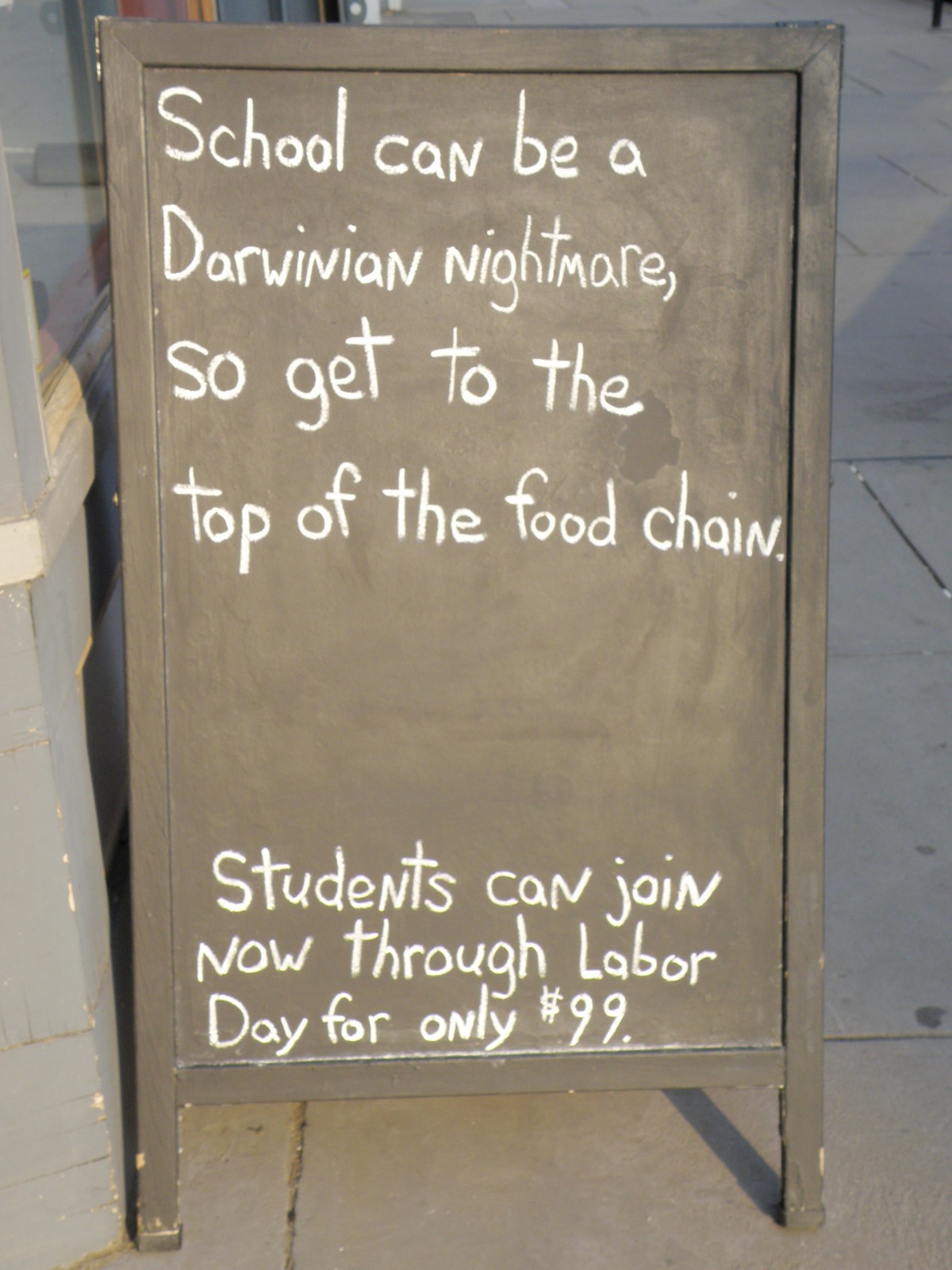The image depicts an A-frame placard sign situated on a gray sidewalk outside a storefront. The storefront features a facade painted in gray or a brownish color, complemented by a glass window. The sign, standing firmly on the sidewalk, has a background in shades of brown, black, or gray and is inscribed with white chalk or chalk paint. The message on the sign reads: "School can be a Darwinian nightmare, so get to the top of the food chain." At the bottom, it further states, "Students can join now through Labor Day for only $99." The surrounding area appears to be devoid of people, cars, or other street elements, emphasizing the sign as the main focus of the image. The sidewalk itself looks a bit dirty, adding an urban feel to the scene.